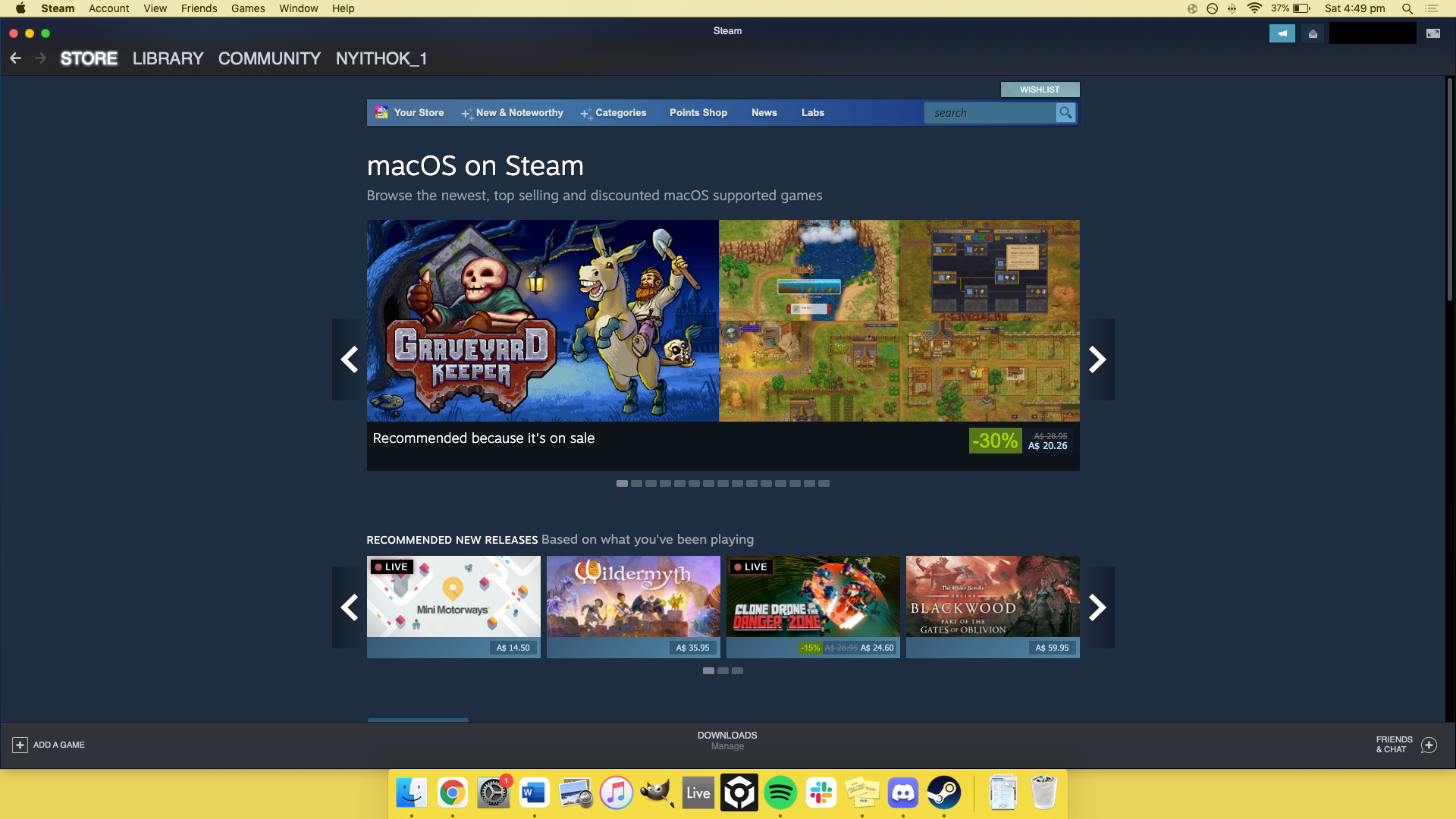This is a detailed screenshot of a computer screen displaying the Steam interface with a navy blue background. At the top of the screen, there's a black strip with three colored dots (red/pink, yellow, and green) on the left side. Below the dots, there is a navigation menu including options labeled "Store," "Library," "Community," and "NYTHOC1." The word "Store" is highlighted in bright white, indicating it has been selected.

Under the navigation menu, there are several sections: "Your Store," "New and Noteworthy," "Categories," "Print Shop," "News," and "Likes." The highlighted section includes a banner for MacOS on Steam, advertising the ability to browse the newest, top-selling, and discounted MacOS supported games. Featured prominently is the game "Graveyard Keeper," which is recommended because it is currently on sale for 30% off. The banner depicts a spooky scene where a man is in a graveyard being pursued by a horse carrying a man with an axe.

Below this, there are additional recommendations for new releases, including "Wild Myth," "Blackwood," "Danger Zone," "Clone Drone," and "Mini Motorways." The entire interface sits against a consistent navy blue backdrop, creating a cohesive visual presentation.